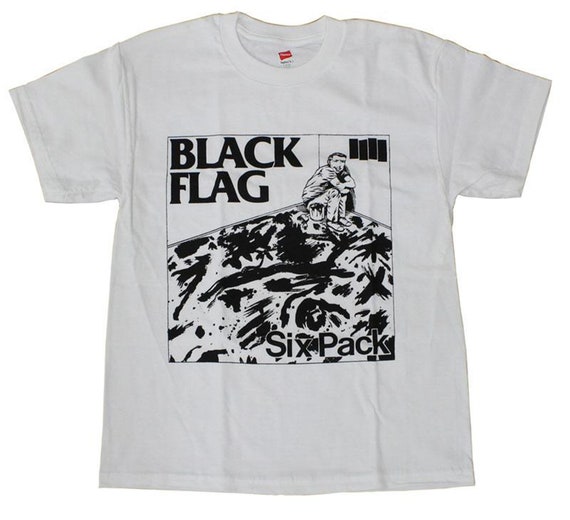This image depicts a white Hanes t-shirt laying flat against a white background, without any human model. The shirt features pronounced vertical creases from being folded into thirds. The predominant graphic on the t-shirt is a black square frame showing a boy, estimated to be around 10 to 15 years old, sitting in a corner with his knees drawn up and his arms folded over them, leaning slightly forward. Above and to the right of his head are four tall, narrow, staggered black rectangles, forming part of the "Black Flag" logo. The words "Black Flag" are prominently displayed in bold black text at the top left of the square, while "Six Pack" is written in smaller black text at the bottom right. The boy is surrounded by black smears on the white floor, denser and more concentrated close to him and sparser further out, suggesting paint strokes, although the exact substance remains ambiguous due to the monochromatic color scheme. The neck of the t-shirt includes a visible Hanes tag, which is white with a red rectangle, positioned somewhat askew. This t-shirt design closely resembles an album cover, capturing a striking and somber scene in stark black and white.